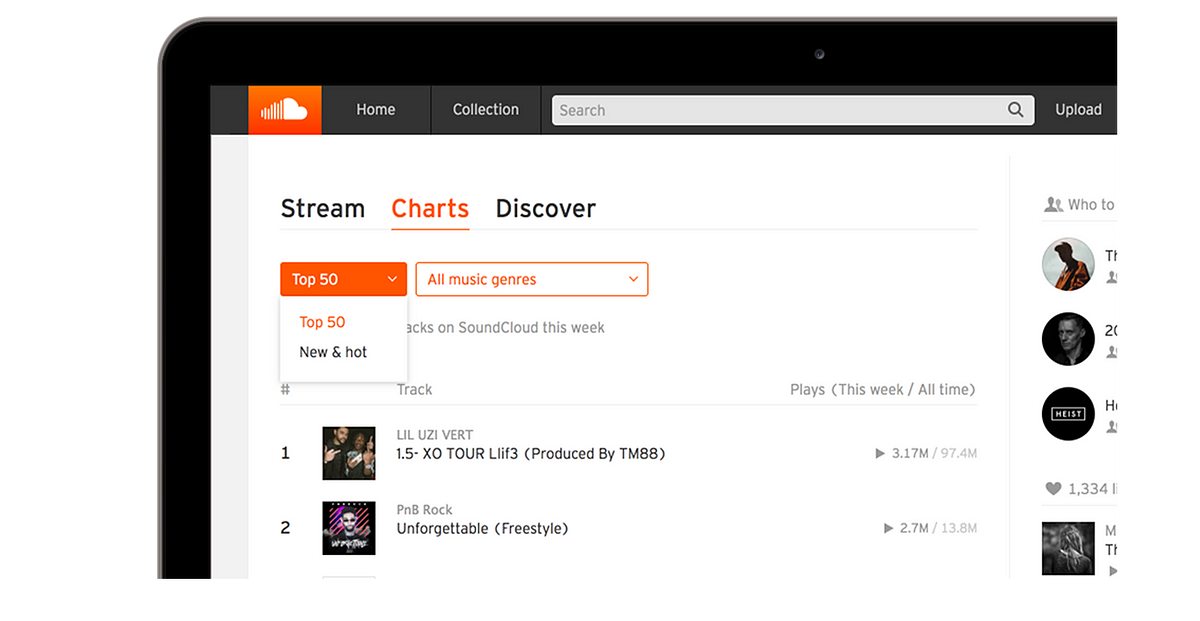A detailed view of a SoundCloud page, showcasing the platform's interface. In the upper left corner, the recognizable SoundCloud logo, an orange rectangle with a white cloud icon, stands out. Adjacent to the logo, on a sleek black background, are the navigation options: "Home" followed by "Collection." Dominating the center of the top bar is a search function, and on the far right, the "Upload" button is prominently displayed. Directly beneath, the tabbed navigation includes "Streams," with the "Charts" tab highlighted in orange, and then "Discover."

A dropdown menu is located below these tabs, with "Top 50" highlighted. Underneath, another selection option reads "New and Hot." The genre selection bar, "All Music Genres," is also highlighted in orange. Beneath this genre bar, columns labeled "Number," "Track," and "Plays" present tracks ranked by popularity for this week and all time. 

The number 1 track features an icon depicting band members, titled "Lil Uzi Vert - XO Tour Llif3," produced by TM88. To the right, a play button is displayed alongside impressive play stats: "3.17m / 97.4m." The second-ranked track shows a picture of an artist wearing sunglasses, titled "PNB Rock - Unforgettable Freestyle," with corresponding play statistics: "2.7m / 13.8m."

Additional icons and partial text are visible in the right-hand column, though their full details are obscured due to the page's cut-off view. The overall layout and design emphasize the ease of navigation and the popularity metrics for trending tracks on SoundCloud.